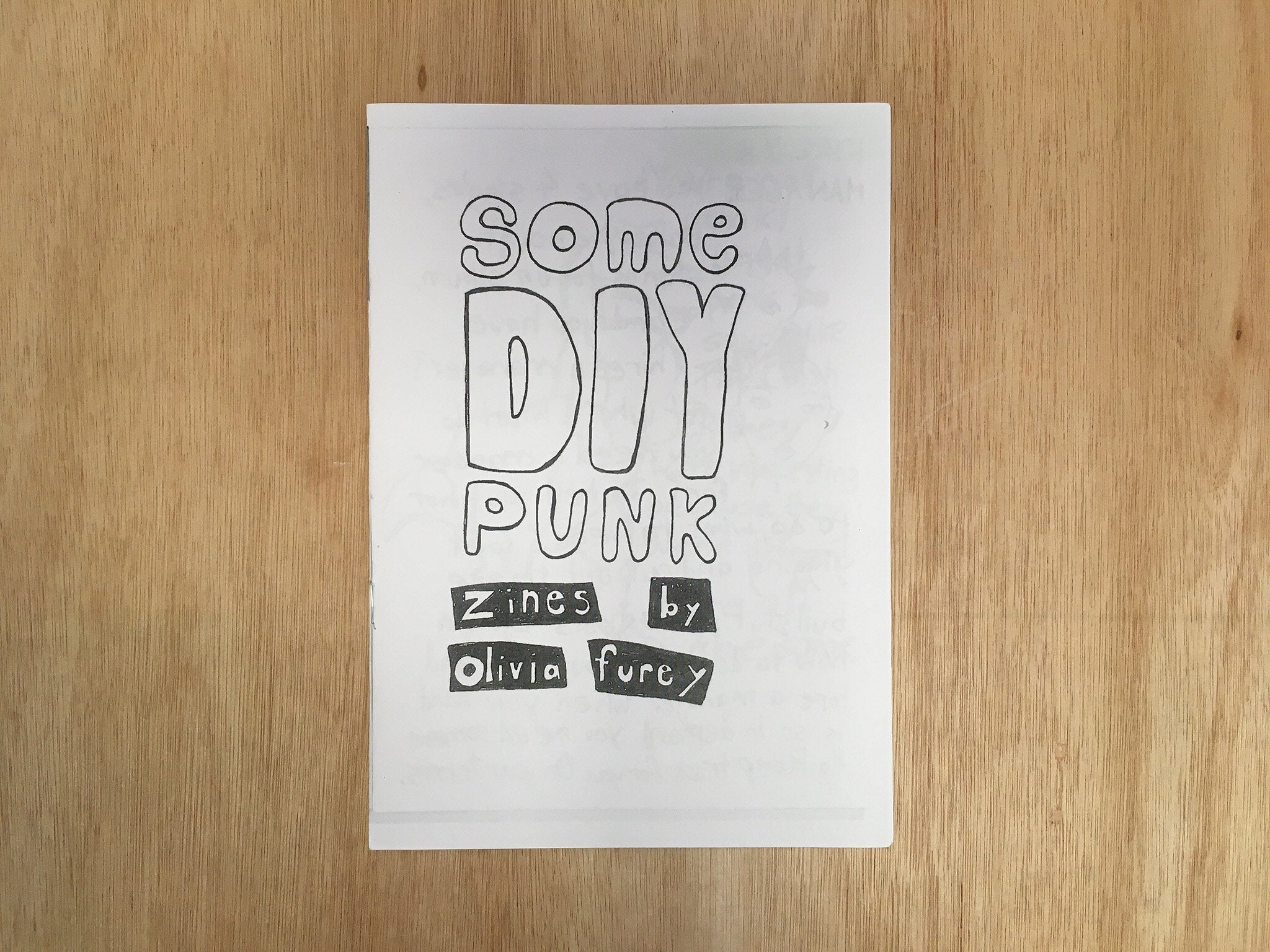A photograph depicts an unpolished, light brown, grainy wooden surface which could be either a tabletop or a wall. On this wooden background, a piece of white paper is placed. The paper features a series of large, black-outlined block letters, creating an unfinished look as if meant to be colored in. At the top, the word "SUM" is outlined in black with white letters, followed by the words "DIY" and "PUNK," also in black-outlined, white letters. Below "PUNK," in a small black rectangular box, the word "ZINES" is written in white text. Another small square-shaped black box below this contains the word "BY," also in white. Further down, two black rectangular boxes each contain a name in white letters: "OLIVIA" and "FUMI." This appears to be an initial graphic design sketch for a cover page, possibly for a child's DIY zine project titled "Some DIY Punk Zines by Olivia Fumi." The rustic texture of the wooden background contrasts with the bold, outlined text on the paper, emphasizing the handmade, punk aesthetic of the project.